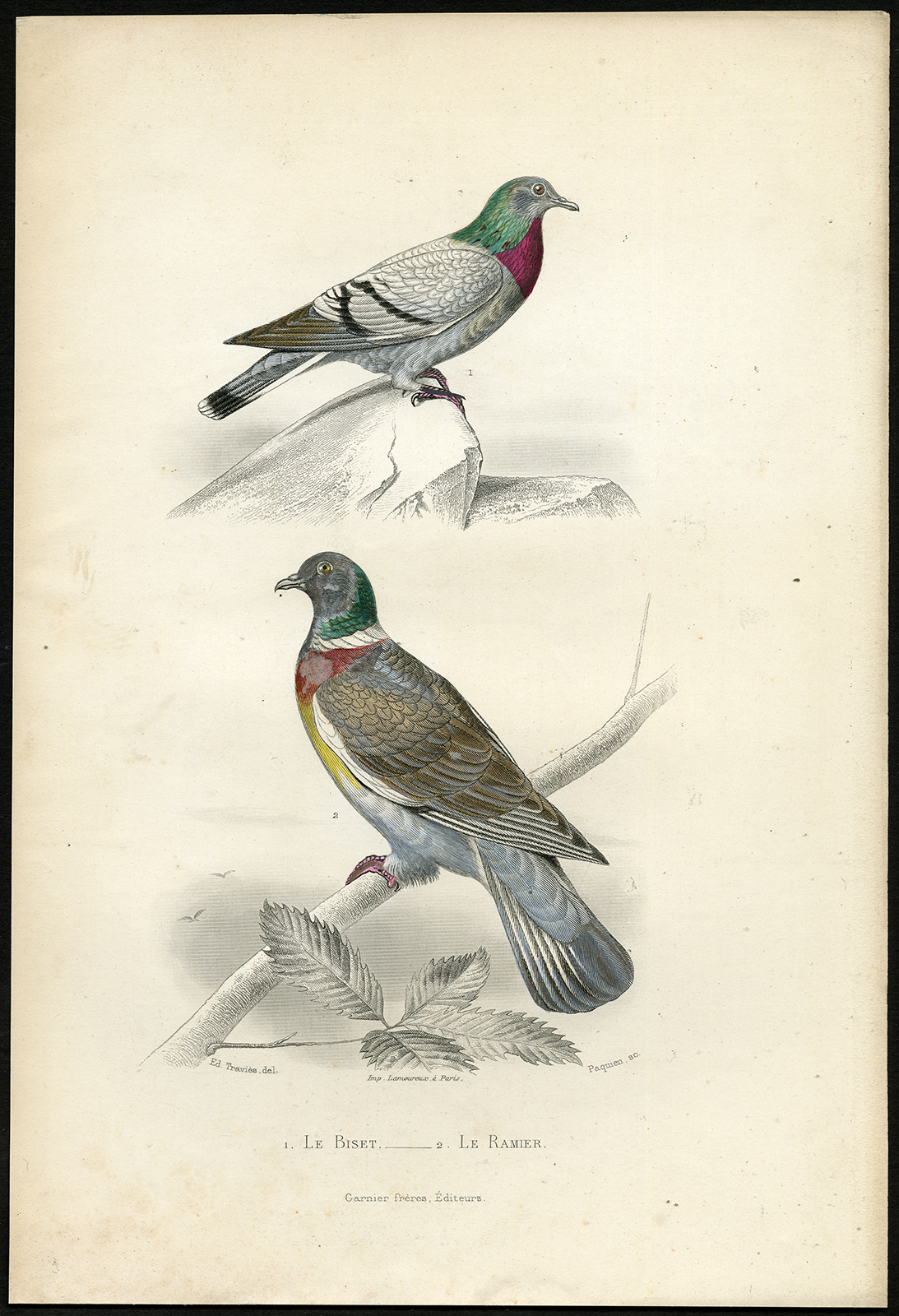This detailed rendering, possibly created with colored pencils, depicts two pigeons in separate, rectangular images, reminiscent of a colored engraving. The top pigeon, shown standing on a rock, features a green head, a red neck, and a white belly. Its wings are white with black stripes and brown tips, and it gazes to the right, presenting its right side. The bottom pigeon, perched on a tree branch with foliage, has a greenish head with gray around the eyes and mouth, a red upper breast, a yellow lower breast, and a light bluish belly. Its brown wings and more brownish tone distinguish it, along with its leftward gaze. The image includes text at the bottom in small uppercase, likely in French, reading "Leigh Bessette Leigh-Romier," suggesting it may be a page from a book.